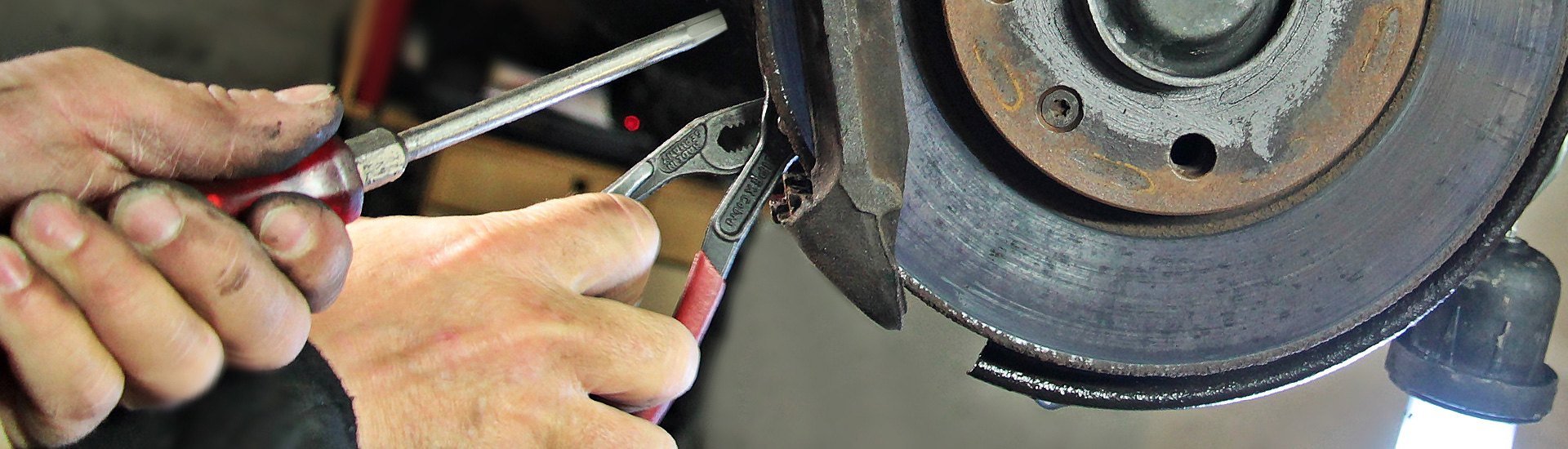This image is a slim, wide, banner-like photograph of a mechanic at work on a car's brake system. On the left side of the photo, two slightly dirty hands, smudged with what appears to be oil, are prominently visible. The mechanic's left hand holds a red-handled screwdriver while the right hand grips a pair of red pliers. The worker, whose arm is clothed in a black long sleeve shirt, is focused on a rust-touched black brake caliper on the right side of the photo. The brake section, detailed by visible screws, is the main focus of the maintenance work. The setting suggests a workshop, possibly with a gray background and a hint of a red tool bench behind the hands.